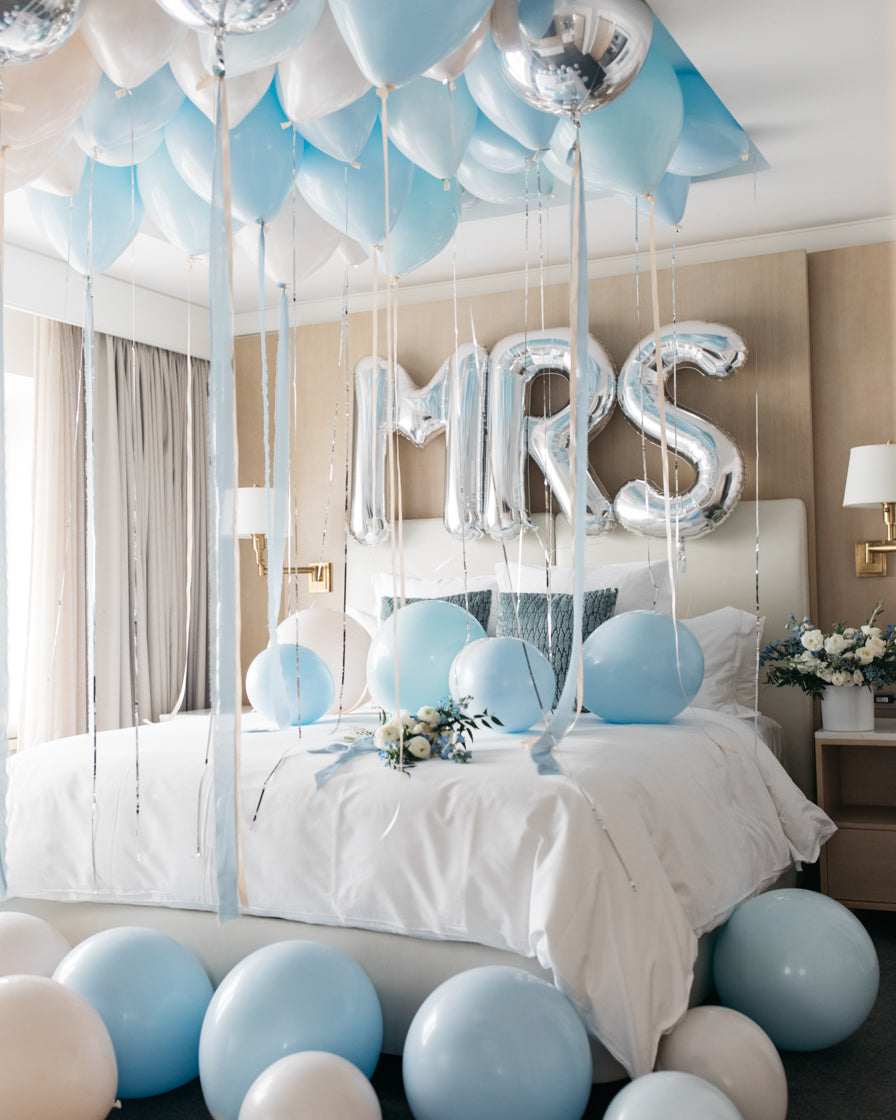This detailed image captures a beautifully decorated bedroom, likely set up for a special celebration such as a birthday, engagement, or bachelorette party. The room centers around a queen-size bed with a white, split headboard. The bed is adorned with white pillowcases featuring a subtle grey pattern, and a white doona cover. Above the bed, gold letters spelling "MRS" suggest a marital occasion.

The room is festooned with numerous balloons in shades of baby blue, white, and a touch of silver. Five balloons rest on the bed—four blue and one white. There are also balloons scattered across the floor, floating along the sides of the bed, and hovering near the ceiling with strings and streams cascading down, likely held aloft by helium.

Adding to the festive atmosphere, a bouquet of white flowers with greenery is placed on the bed, accompanied by another flower arrangement on one of the side tables flanking the bed. The nightstands host dual lamps with white shades and silver accents, which are mounted on the wall.

The room itself features a white ceiling, soft brown walls, and a mid-brown carpet. The window to the left is dressed in bone-brown curtains with white trim around the architraves. The overall aesthetic and meticulous decoration give the impression of a luxurious hotel room prepared for joyous festivities.